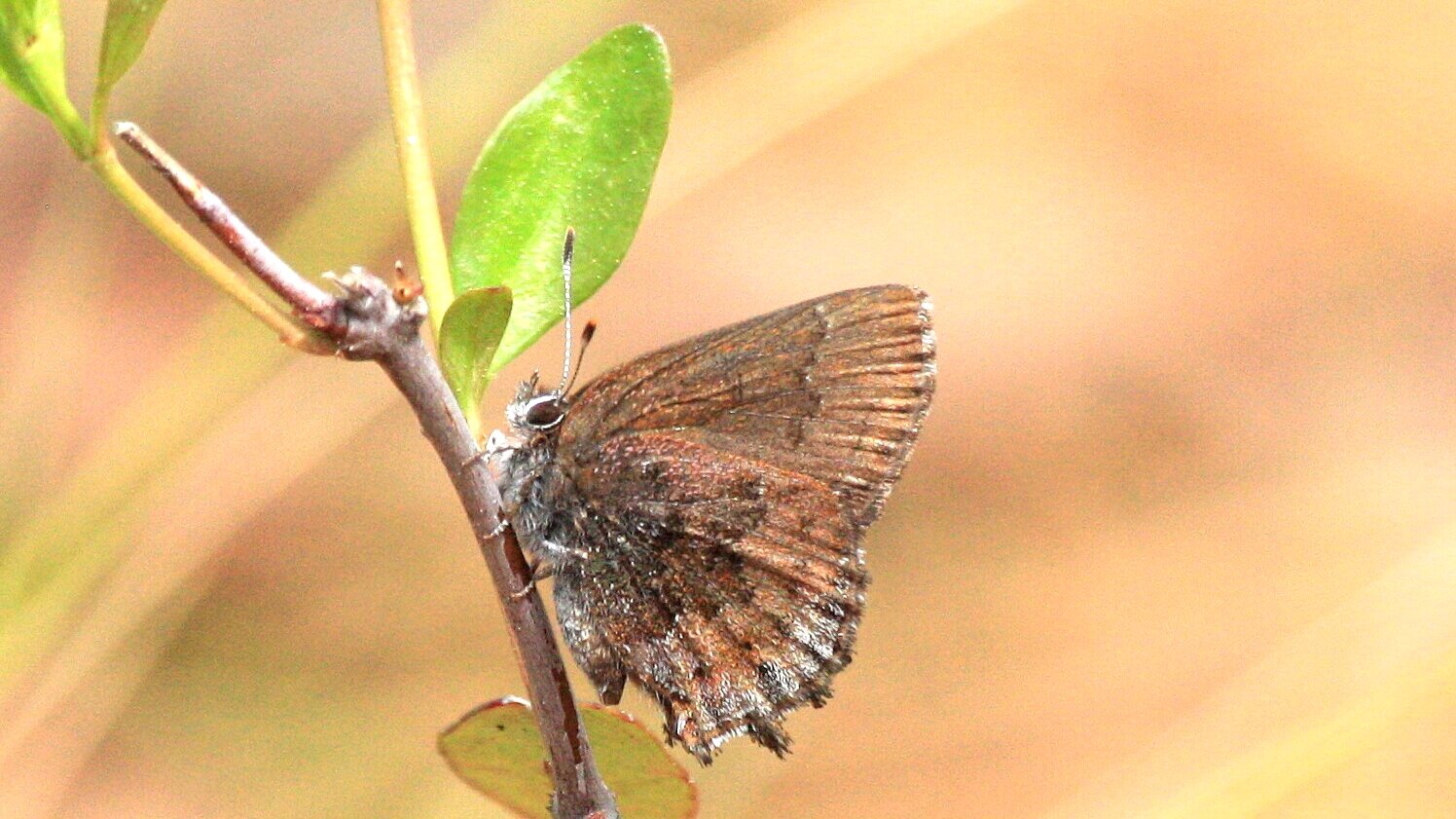In this close-up, horizontally cropped photograph, a moth is perched on a slender twig that sprouts fresh, bright green leaves. The moth itself, sitting slightly left of center, boasts a furry appearance with large black eyes and fuzzy antennae. Its wings display a blend of muted, rust-brown colors accented by patches of white and black, with slightly elongated tufts at the bottom edges. The background of the image is heavily blurred, featuring subdued pastel hues of peach, yellow, and pink, along with some streaks of green and white. The overall tone of the photograph is light and aesthetically pleasing, capturing a delicate moment in nature with a soft-focus effect enhanced by a subtle red tint, giving the image a gentle, serene atmosphere.